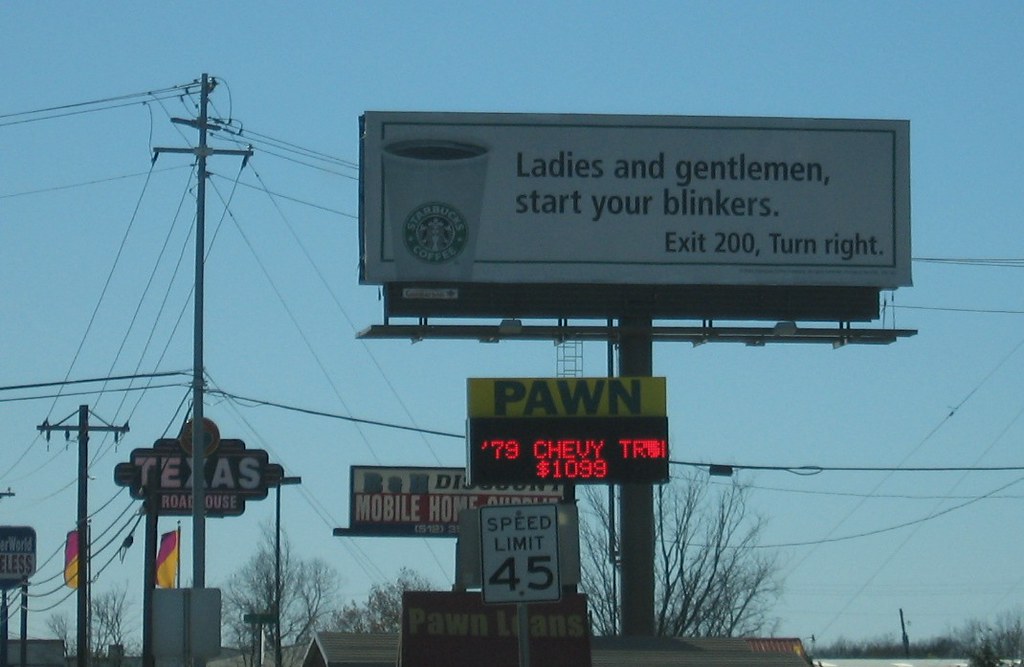The photograph captures an urban streetscape dominated by various signs, poles, and power lines. Central to the image is a prominent billboard featuring an advertisement for Starbucks with the text, "Ladies and gentlemen, start your blinkers. Exit 200, turn right," alongside an image of a Starbucks coffee cup set against a white background. 

Below and behind the billboard, there is an array of business signs. Directly beneath it is a large sign for a pawn shop displaying "Pawn" in bold, with an LED message reading "79 Chevy TR $1,099" beneath it. This sign partially obscures a "Speed Limit 45" sign, which stands slightly ahead of another sign for the pawn shop offering "Pawn Loans."

In the backdrop, a "Mobile Home" sign appears, although its details are somewhat hidden by the preceding signs. Above all of these, the recognizable signage for a Texas Roadhouse peeks through, with a utility pole inconveniently bisecting the "X" in "Texas."

Interwoven through the scene are numerous power poles and power lines, contributing to the urban feel with their tangle of cables. In the distance, autumn-hued trees add a touch of natural color to the landscape.